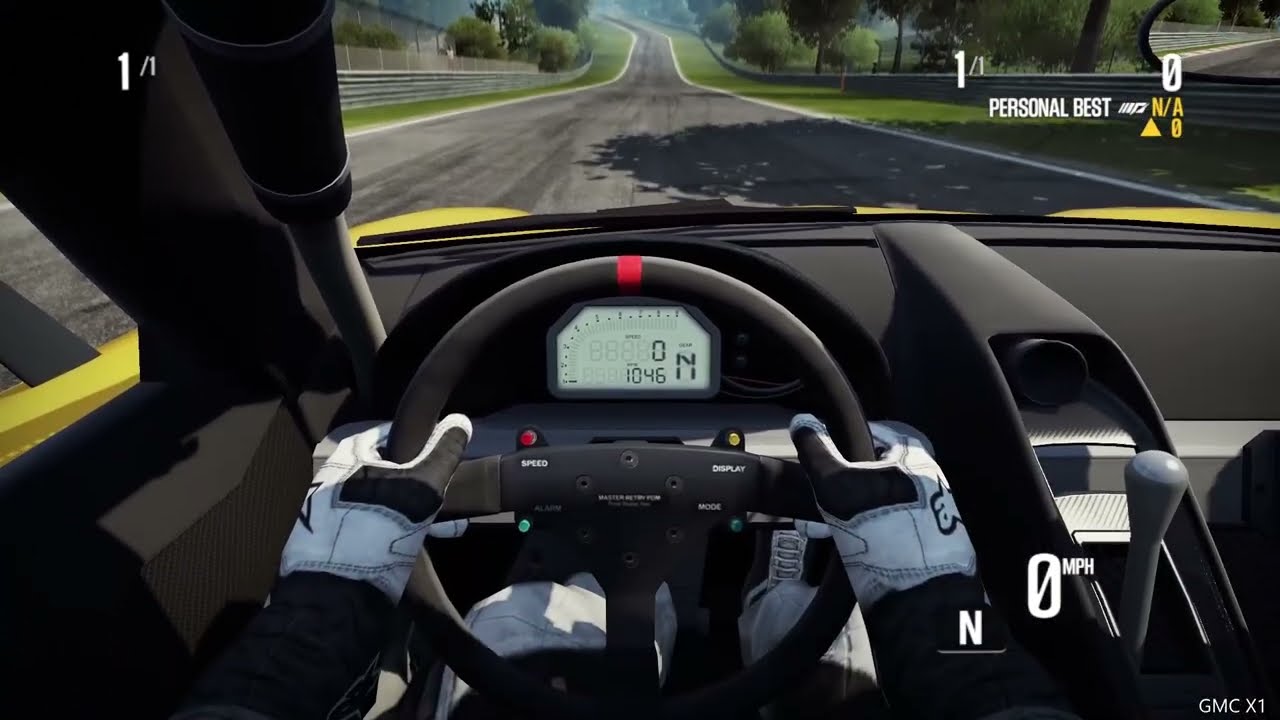The image is a detailed screenshot from a first-person perspective racing video game. The viewpoint is from inside the vehicle, showing a black steering wheel gripped by two gloved hands—white and black gloves are worn by the driver, whose attire includes white pants and a black jacket. On the right, under the steering wheel, there's a visible gear shifter. The dashboard displays a speedometer and several dials, with animated overlays indicating "0 miles per hour," a large "N" for neutral, "personal best" in the top right, and "1 of 1" in the upper left. Through the windshield, an open paved racing track can be seen, flanked by green grass, trees, and fencing on both sides. The track runs straight into the center before curving slightly to the left. The overall setting gives the feel of high speed and precision driving in a race car.